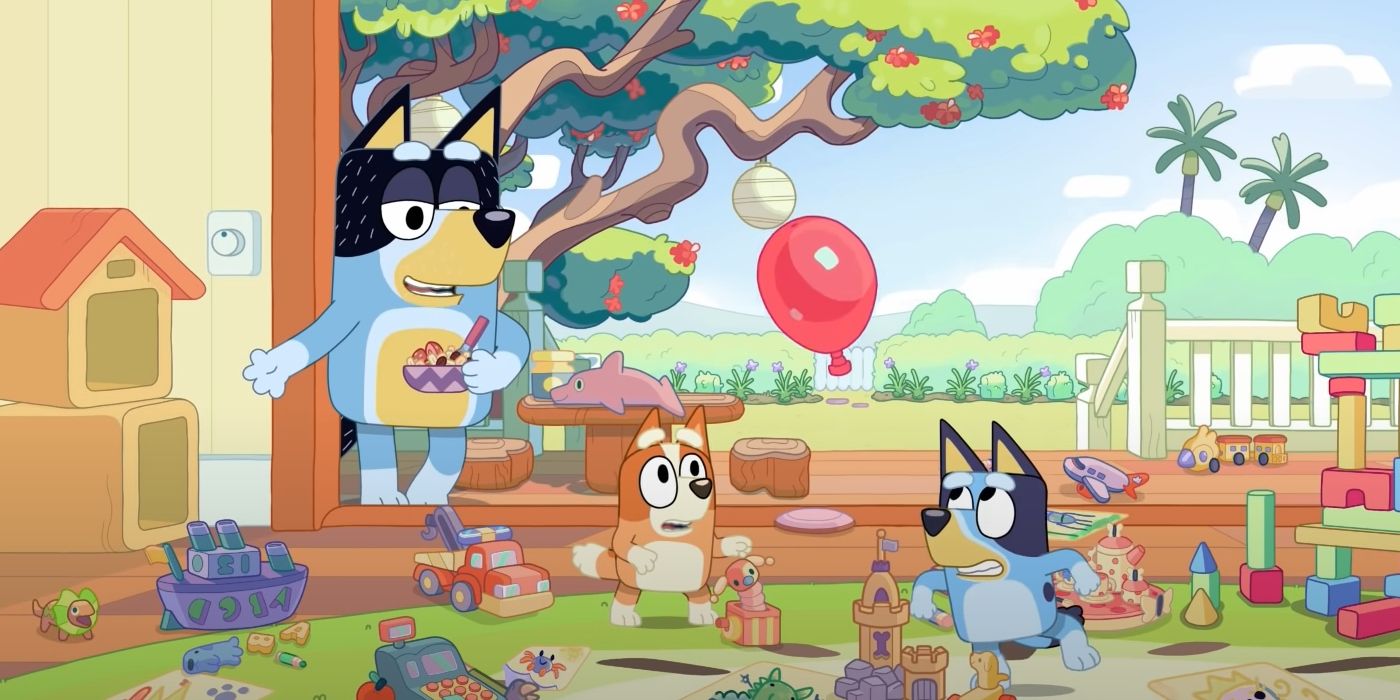This is a vibrant scene from the popular children's TV show "Bluey." The background features a blue sky with fluffy white clouds, a green hill, and an array of palm trees and green bushes. A notable tree with red flowers and hanging white ball-like objects stands out among the flora. In the foreground, various colorful toys, including cars, trucks, boats, castles, planes, and blocks, are scattered on the green grass. 

Central to the scene are three anthropomorphic dogs. The largest, Bluey, stands prominently holding a mixing bowl, possibly containing ice cream or food, with a spoon sticking out. Bluey has a blue and black fur coat with white eyebrows and gray eyelids, and extends his right hand towards something resembling a doghouse. 

To Bluey's left is a brown and white dog with white eyebrows, standing on its hind legs, gazing upwards with a serious expression. On Bluey's right, a smaller dog similar in appearance to Bluey—blue and gray with white eyebrows and black nose—also stands on its hind legs, looking up intently. The scene exudes a blend of playfulness and seriousness, typical of the engaging and wholesome adventures in "Bluey."